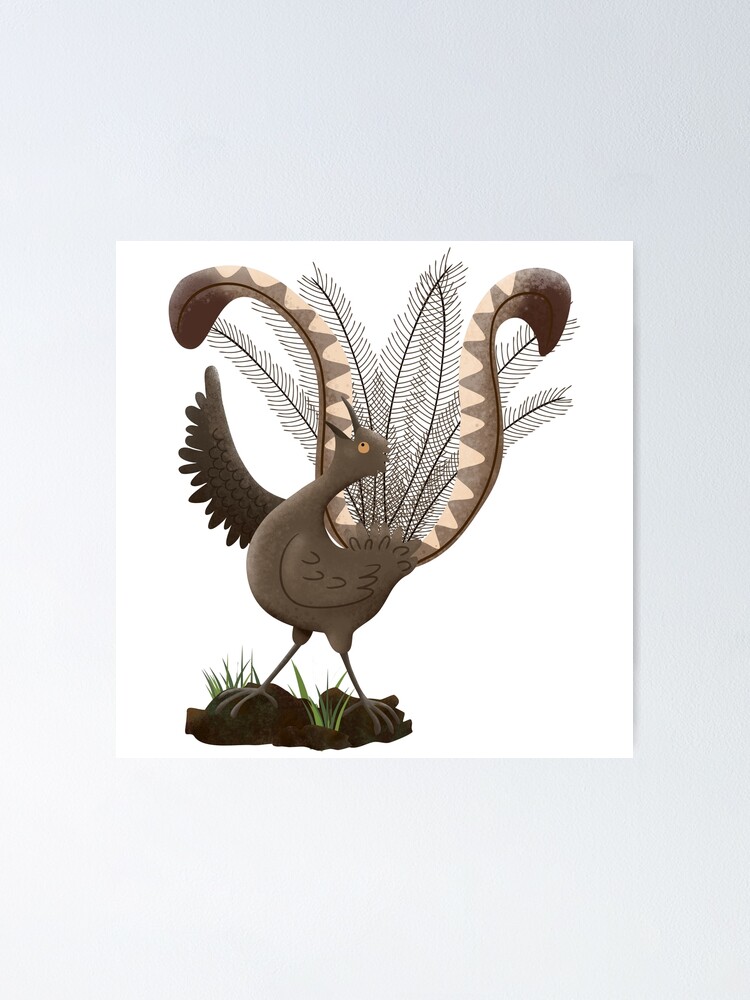In the image, a bird with a darker plumage is captured in a vulnerable position. The bird's beak is pointed sharply upwards, slightly open as if snapping at the air. A noticeable light shadow, cast by the bird, spreads across the ground, adding depth to the scene. Despite its precarious posture, the bird shows no sign of rabies or severe illness. The overall composition and lighting highlight the bird’s delicate state against its contrastingly dark feathers.